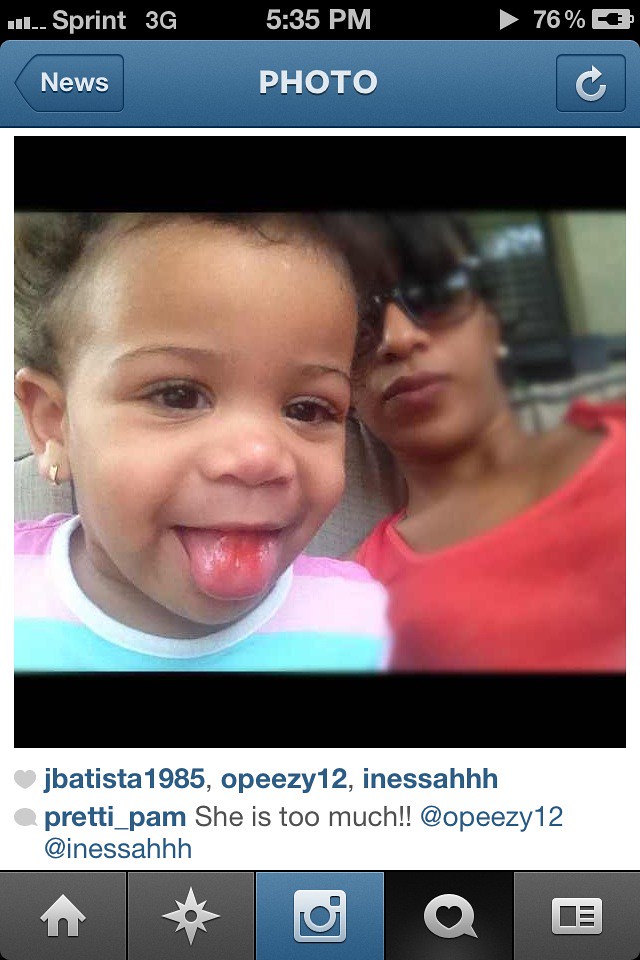This image is a detailed screenshot from an iPhone displaying a moment captured on Instagram. The top of the screen shows it is 5:35 p.m., with a 75-76% battery charge and Sprint 3G as the network indicator. The main feature of the photo depicts a young girl and her mother. The little girl, dressed in a pink, white, and teal striped shirt with a small gold earring in her ear, is closest to the camera, smiling broadly with her tongue sticking out, showing a red stain that might be blood or candy dye. Her mother, positioned slightly behind, is wearing a red tank top and tinted sunglasses, maintaining a neutral expression. The Instagram interface further adds detail, showing likes from users "Jay Batista, 1985," "OPZ12," and "NESSAAH," and a comment from the user "Pretty Pam" saying, "she is too much" directed at "OPZ12." The lower section of the interface includes navigation buttons typical of old Instagram, such as Home, Navigation, and a central Instagram button, along with sections for likes and comments, culminating in a nostalgic view of an older social media post.